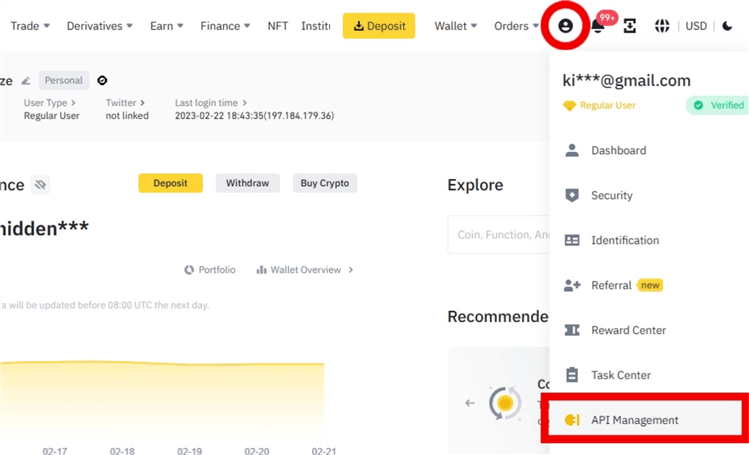This cropped screenshot captures a segment of the Binance homepage. On the right side of the image, there is a vertical panel with a white background, displaying a dropdown menu of user information. At the top right corner, a red circle highlights the profile icon, indicating where users need to click to access the dropdown menu. Below the profile icon, the dropdown lists various pieces of information starting with the user’s sign-in details. 

Prominently featured is a gold diamond icon with bold gold text indicating a "Regular User" status, followed by a "Verified" label. The menu contains several options in a vertical arrangement, concluding with "API Management," which is enclosed in a red box for emphasis.

On the left side of the image, there is a partial view of the main page. Despite being cropped, you can identify the navigation options such as "Trade," "Derivatives," "Earn," "Finance," "NFT," and "Institution." Adjacent to these options, a large yellow "Deposit" button is visible. To the right, there are dropdown boxes labeled "Wallet" and "Orders." Below these options, a gray horizontal box displays user-specific information, including user type (Regular User), Twitter status (not linked), and the last login time, which is highlighted in black text.